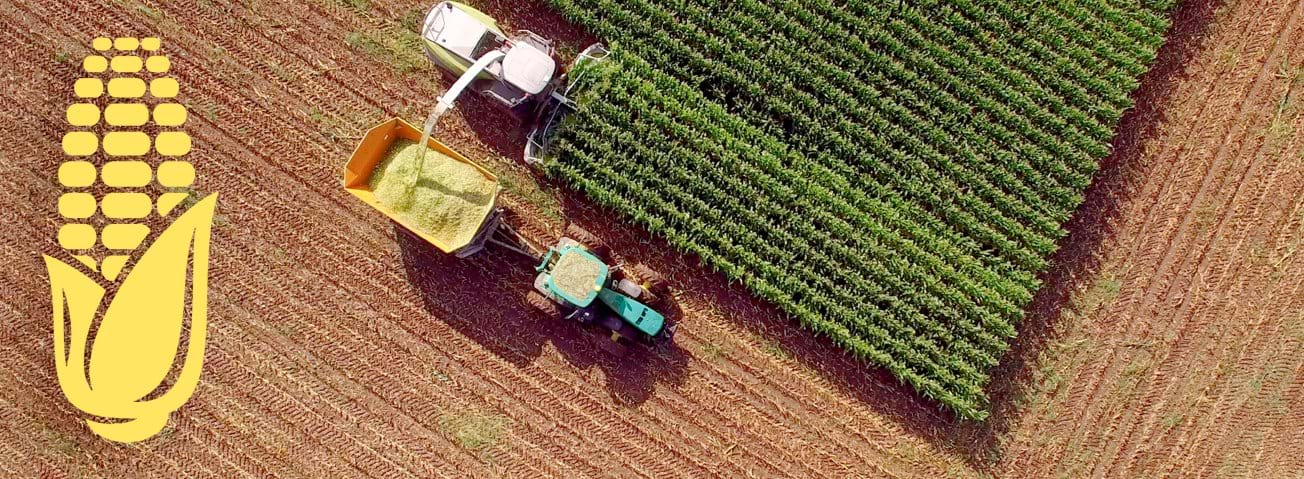In this horizontally oriented, rectangular aerial photo, we observe a bustling farm field centered around the activity of harvesting corn. Dominating the scene is a white combine equipped with a distinctive pipe, busily collecting eight rows of vibrant green corn at a time. This combine discharges its harvest into a yellow wagon pulled by a green tractor traveling alongside. The outer edges of the field, already harvested, reveal a patterned beige dirt adorned with tire tracks and brown stubble from the cut corn. Adding to the agrarian essence, a large, cartoon-like corn icon appears on the left side of the image, featuring yellow kernels and green leaves. This icon seems to be part of an advertisement promoting a corn product.